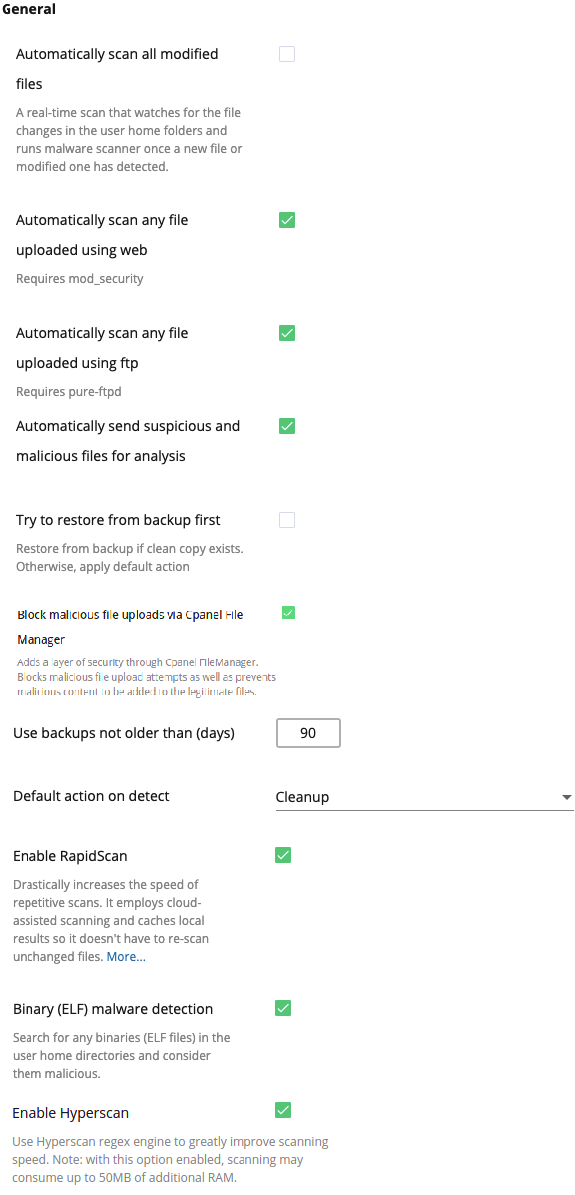This is a detailed caption for the described image:

"A screenshot of the admin interface from Immunify360 showcasing the 'General' section at the very top left, highlighted in bold black. The section contains multiple rows, each consisting of a title, a brief description, and an accompanying checkbox. Some checkboxes are marked in green, indicating they are active, while others remain unchecked. The rows are as follows:
1. 'Automatically scan all modified files' - Unchecked.
2. 'Automatically scan any file uploaded using web' - Checked in green.
3. 'Automatically scan any file uploaded using FTP' - Checked in green.
4. 'Automatically send suspicious and malicious files for analysis' - Checked in green.
5. 'Lock malicious files uploaded to storage' - Checked in green.
6. 'Enable rapid scan' - Checked in green.
7. 'Binary ELF malware detection' - Checked in green.
8. 'Enable hyperscan' - Checked in green.
The remaining rows, though not listed, are unchecked. The entire interface is set against a white background, providing a clean and clear visual layout."